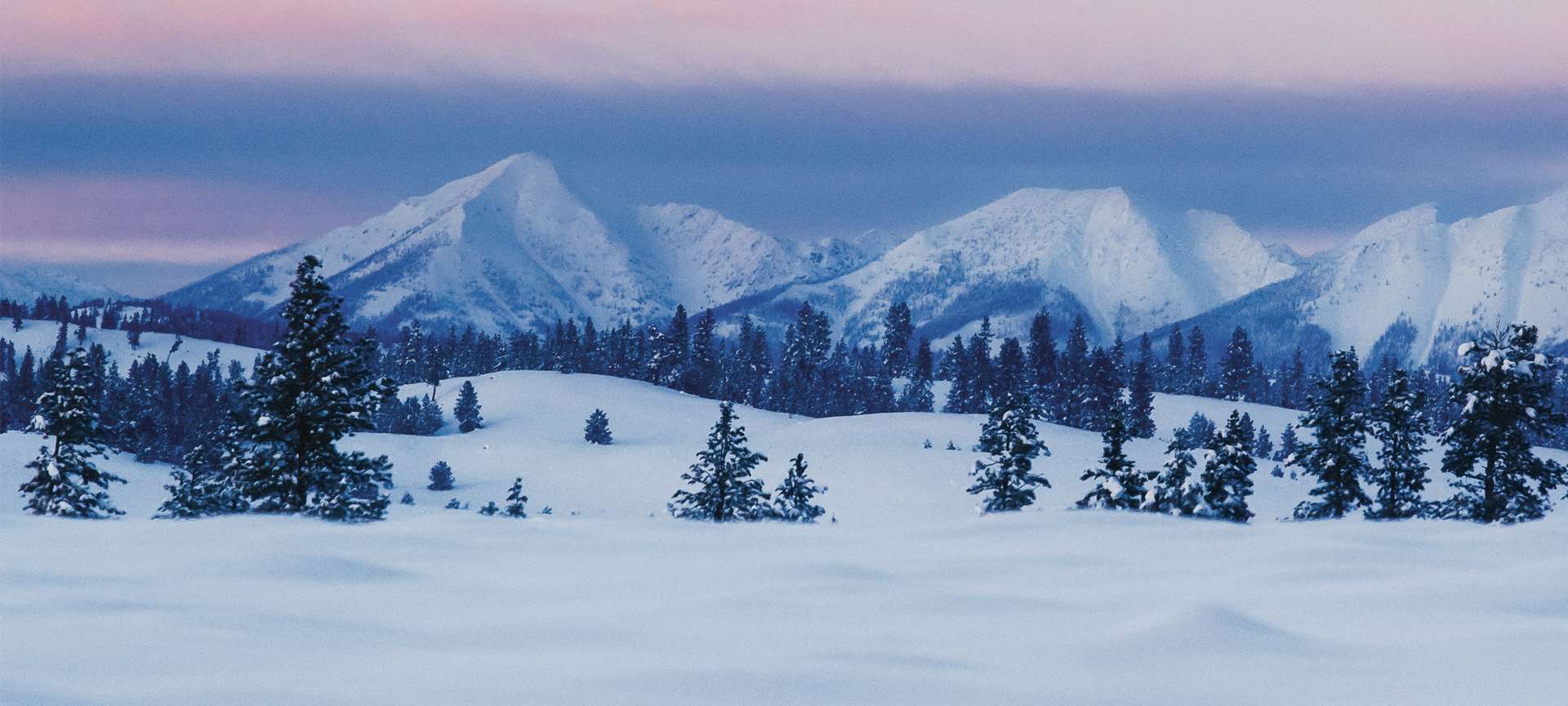The photograph captures a breathtaking snowy landscape featuring a vast expanse of pristine white snow extending into the horizon. In the foreground, clusters of tall pine trees, with dark, snow-covered needles, are partially buried under several feet of snow, only their tops peeking out. These trees appear in layers, with some closer to the foreground and others receding into the distance, creating a sense of depth and scale. Rolling hills of snow lead up to a line of towering, snow-capped mountain peaks in the background, which are highlighted by a dramatic sky filled with layers of pink and gray hues. The base of the mountains shows hints of grayish rock beneath the dense snow, enhancing the rugged beauty of the scene. Overall, the image portrays a serene yet majestic winter wonderland, with rich textures and contrasting colors that emphasize the depth and grandeur of the natural setting.